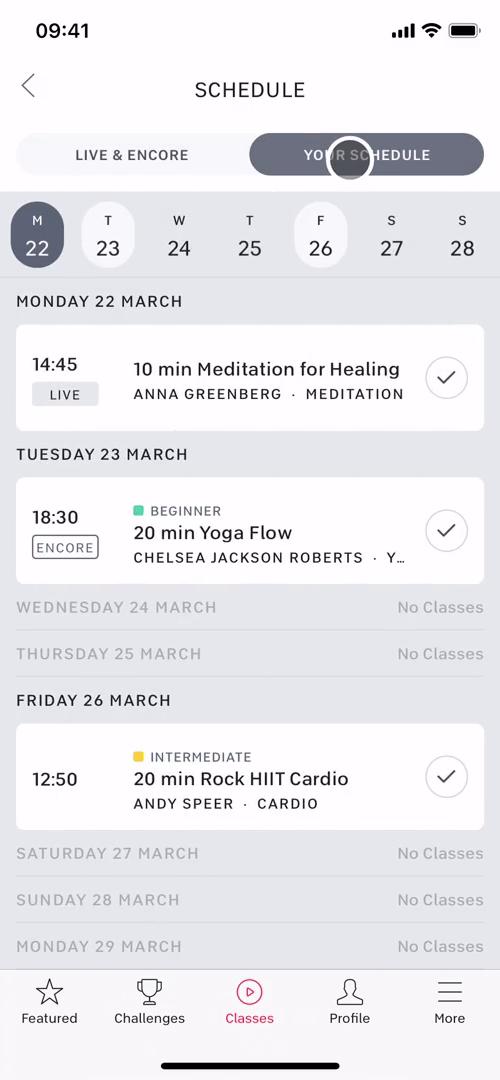This image is a screenshot from a mobile app, likely on an iPhone, displaying a calendar interface. The background is light, and the layout is taller than it is wide. The color scheme is predominantly monochromatic, featuring shades of white, light gray, dark gray, and black text. At the top of the screen, the word "Schedule" is prominently displayed. Below this heading, the app shows the week ahead, listing the days in abbreviated form: M (Monday), T (Tuesday), W (Wednesday), T (Thursday), F (Friday), S (Saturday), S (Sunday). The week starts with Monday, the 22nd, and continues through Sunday, the 28th. 

Beneath the weekly overview, more detailed schedules are provided. For Monday, March 22nd, there is a scheduled "10-minute Meditation for Healing" with Anna Greenberg at 14:45. Following this, the schedule for Tuesday, March 23rd features a "20-minute Beginner Yoga Flow" class with Chelsea Jackson Roberts at 18:30, marked as an encore session. The next visible entry is for Friday, March 26th, detailing a "20-minute Rock HIIT Cardio Workout" with Andy Speer at the intermediate level, set for 12:50.